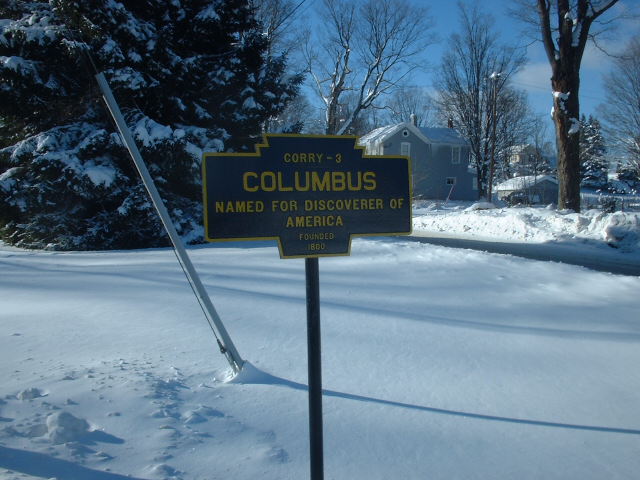In this photograph taken on a snowy day, the landscape is dominated by a vividly snowy expanse. Front and center stands a prominent sign that reads "Corrie-3 Columbus, named for Discoverer of America, founded 1880," though the smaller text may appear unclear. The sign itself is rectangular with a banner shape on top, featuring bold yellow text on a dark background, outlined in gold and mounted on a black pole. The backdrop reveals a blue sky peppered with a few clouds. On the left side in the foreground, a large evergreen tree is laden with a heavy load of snow on its branches, providing a striking contrast against the clear sky. To the right, the barren branches of deciduous trees peek through the snow. In the distance, across what seems to be a field or shoveled driveway, stands a gray house covered in snow, complete with two chimneys. Nearby, a utility pole with visible cables is partially hidden by a hollow gray housing, adding a touch of industrial detail to the otherwise natural, wintry scene.